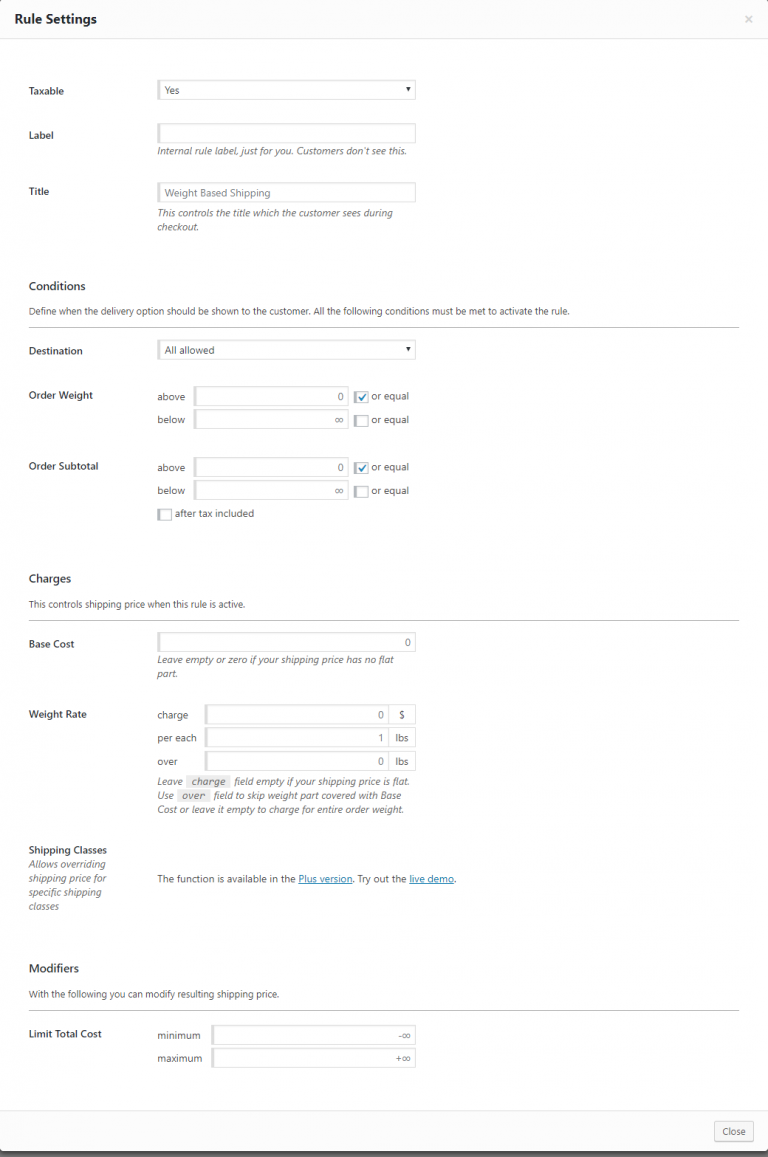**Detailed Caption for Image:**

The image depicts a settings screen with a predominantly white background. At the top, there's a gray header section labeled "Rural Settings" in black text. Below this header, various customizable options are presented.

1. **Settings Options**:
   - **Editable Field**: To the right is a drop-down menu, with "Yes" selected. Below it is an empty field labeled "Internal Rule Label" with the note that customers won't see this label.
   - **Title**: The field is titled "Weight-Based Shipping" and contains an empty text box pre-filled with the placeholder "Weight-Based Shipping." A description underneath reads: "This controls the title which the customer sees during checkout."
   
2. **Conditions Section**:
   - A gray description states: "Define when the delivery option should be shown to the customer. All the following conditions must be met to activate the rule."
   - Below the gray divider line:
     - **Destination**: Labeled "All Allowed" with a drop-down menu.
     - **Order Weight**: Contains two segments; the top segment has a text box with "0" and a blue-checked checkbox labeled "are equal." The bottom segment contains an infinity symbol in a text box and an unchecked checkbox.
     - **Order Subtotal**: Mirrors the "Order Weight" layout with text boxes. Below it, there's an additional empty white text box labeled "after tax included."

3. **Charges Section**:
   - Described as controlling the shipping price when the rule is active.
   - Divided by a gray line:
     - **Base Cost**: An empty text box with "0" and descriptor text advising to leave it empty or "0" if there's no flat shipping cost.
     - **Weight Rate**:
       - Initially labeled "Charge Per Each" with empty checkboxes.
       - Default placeholder: "0 dollars per each" and "over (lbs)."
       - Below is a descriptive note indicating to leave the charge field empty if the shipping price is flat or to charge for the order's total weight if not.

4. **Shipping Classes**:
   - The description indicates it allows for overriding the shipping price for specific shipping classes.
   - A note to the right reveals that this function is available in the Plus version, with links labeled "Try Out the Live Demo" and "Plus Version of Live Demo" in blue text.

5. **Modifiers Section**:
   - Description states: "With the following, you can modify results shipping price."
   - Includes a gray line followed by "Limit Total Cost" with two text boxes labeled "Minimum" and "Maximum." The minimum field is filled with "-0.00" and the maximum with "+0.00."

At the bottom right of the screen, there's a gray section containing a "Closed" button.